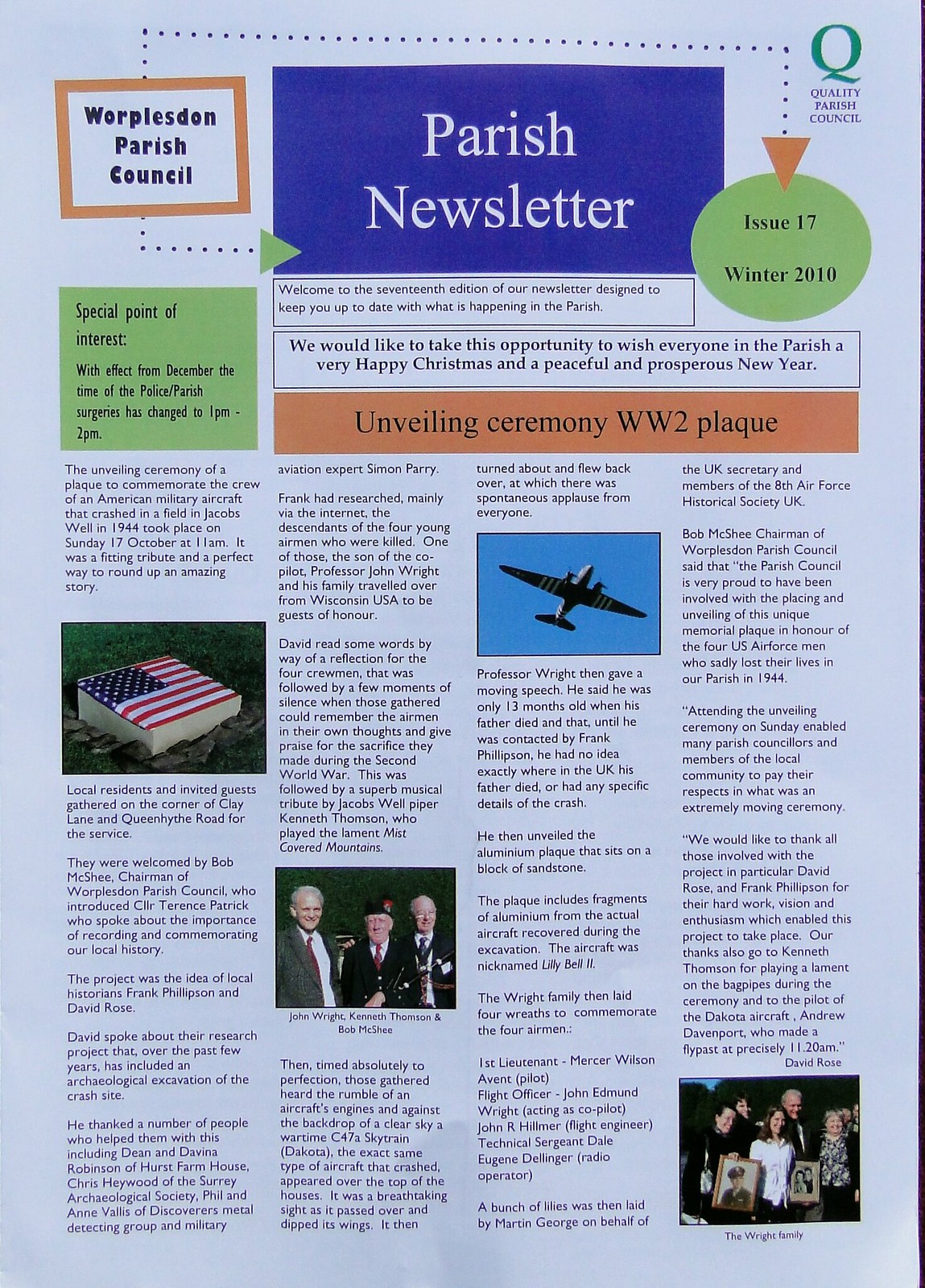The image is a photograph or scan of a detailed parish newsletter with a grayish blue background. At the top, a prominent blue box features the title "Parish Newsletter" in large white font, centered between the left and right sides. To the left within this blue box, there is an orange-outlined box with "Warplizden Parish Council" written in black. On the right, a green circle denotes "Issue 17 Winter 2010" in black lettering. Below, several black-outlined boxes contain additional information in black writing. A special interest is highlighted in a green box to the left: "With effect from December, the time of the police/parish surgeries has changed to 1 p.m. to 2 p.m." Centrally placed is an orange rectangle titled "Unveiling Ceremony World War II Plaque" in black writing. The bottom third of the newsletter contains multiple paragraphs and several photographs interspersed throughout. On the left, an image depicts a grave with an American flag. Above this, a photo showcases a plane in the sky. Additional images, located towards the bottom right and left, feature individuals in suits attending memorial events. The newsletter also extends holiday wishes to the parish community, encouraging a happy Christmas and a prosperous new year.